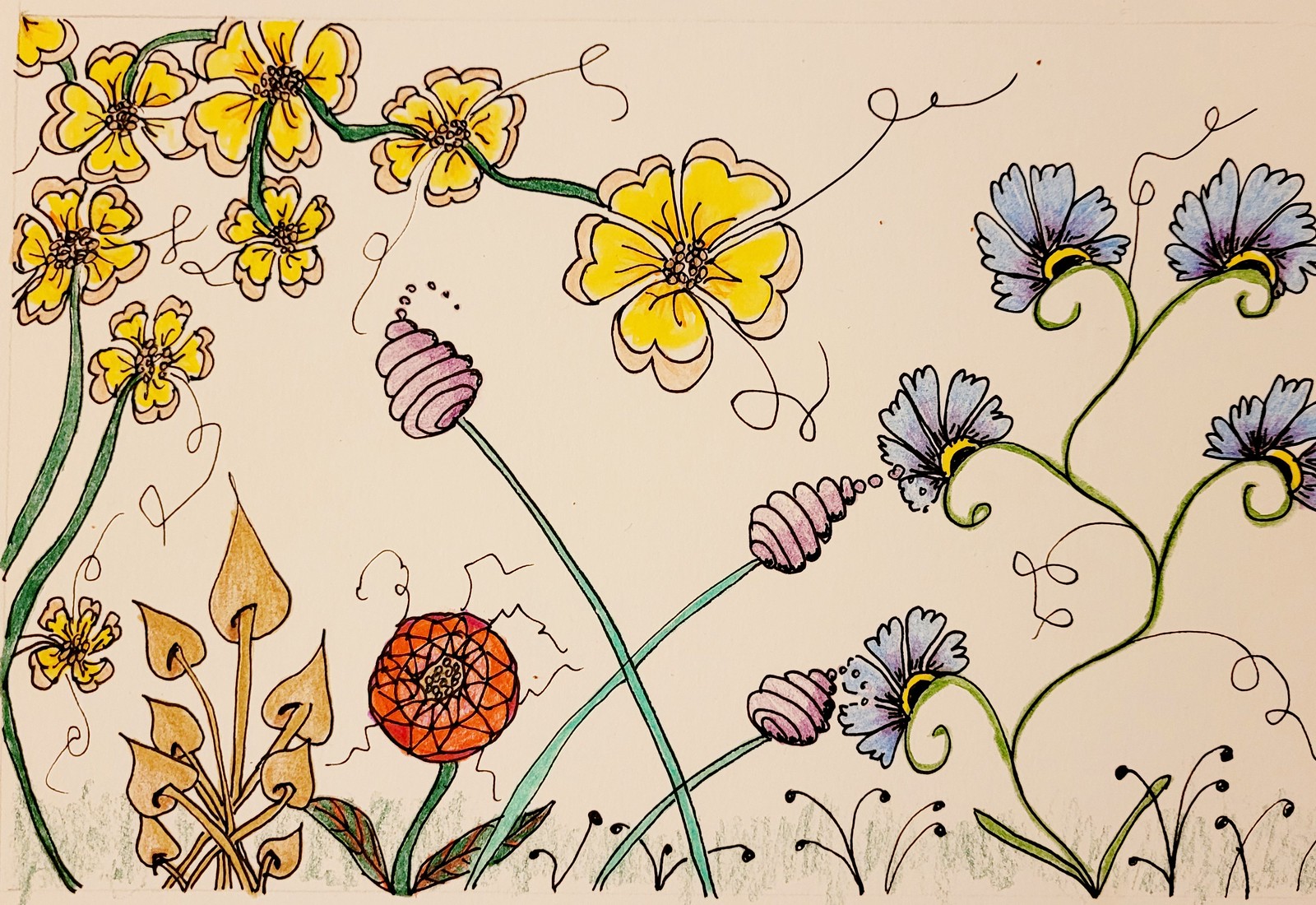The image, digitally scanned for high resolution, features a detailed and colorful nature scene, most likely created with a mix of ink and colored pencils on a creamy, beige background. Dominating the upper left section are several yellow flowers with heart-shaped petals that fade to pink at the edges, connected by greenery resembling a vine. Moving rightward, there's a light brown plant shaped like spades, adjacent to a vivid orange and red marigold. In the center, a trio of purple flowers resemble honeycombs or beehive patterns, and to their right, a light blue flower completes the arrangement. Scattered throughout are various leaves and curly plant tendrils, adding to the intricate floral composition.